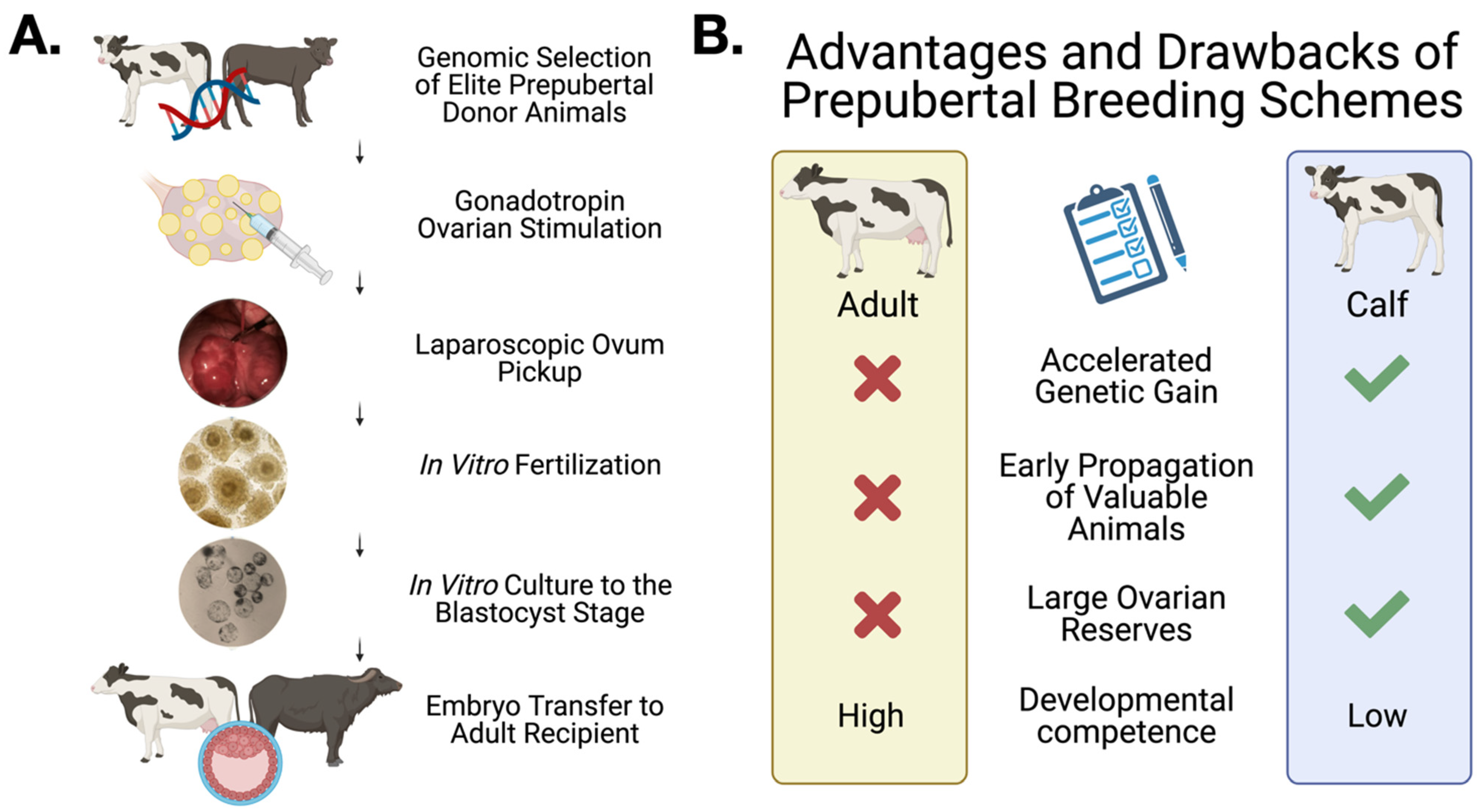The image is a detailed graph presented in a landscape orientation, divided into two labeled halves, A on the left and B on the right. The top left corner shows "A" in bold black text, with two images of cows underneath— a black-and-white cow on the left and a gray cow on the right. The flowchart next to these images reads "Genomic Selection of Late Pre-Pubertal Donor Animals," followed by sequential stages connected by downward arrows: "Gonadotrophin Ovarian Stimulation," "Laparoscopic Ovum Pickup," "In-vitro Fertilization," "In-vitro Culture to the Blastocyte Stage," and finally "Embryo Transfer to Adult Recipient." Each stage is accompanied by corresponding icons, including a chromosome artwork in red and blue and an image of a syringe. 

The right half of the image, labeled “B” at the top in large black letters, is dedicated to listing the "Advantages and Drawbacks of Pre-Pubertal Breeding Schemes." This section contrasts adult cows and calves, marked by X's and green check marks, respectively. The four points highlighted are "Accelerated Genetic Gain," "Early Propagation of Valuable Animals," "Large Ovarian Reserves," and "Developmental Competence," with the last point noting high competence for adults and low for calves.